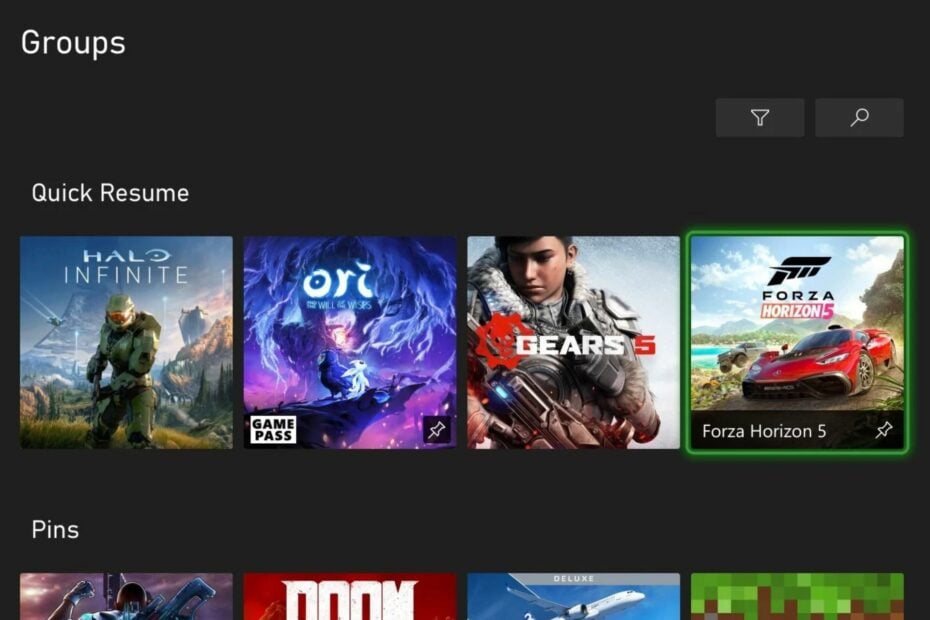The background image showcases multiple game thumbnails arranged aesthetically from top left to bottom right, each adorned with distinct visuals and texts:

1. **Top Left:**
   - **Games Overview:** A grey square with a filter icon and a magnifying glass, accompanied by white text reading "Quick Resume."
   
2. **Halo Infinite:**
   - **Visuals:** Shows Master Chief armed with a rifle.
   - **Background:** Clear blue sky and green ground, with spaceships hovering in the distance.
   
3. **Ori and the Will of the Wisps:**
   - **Main Characters:** Displays Ori, a ghostly creature, standing next to an owl.
   - **Setting:** Enchanted forest with an ethereal tree in the background.
   
4. **Gears 5:**
   - **Character:** Features a figure with a fuzzy neck and armor, ready for combat.
   
5. **Forza Horizon 5:**
   - **Vehicle:** Depicts a sleek red sports car against a vibrant backdrop.
   - **Text:** White text reading "Pins."
   - **Additional Visuals:** Shows a person with their fist raised, clad in a glove, with a rifle in the backdrop and a purple-tinged sky.
   
6. **Doom:**
   - **Title Text:** White text stating "Doom."
   - **Background:** Dominantly red with a grey top section labeled "Deluxe."
   - **Additional Elements:** There is a hint of blue in the background.
   
7. **Minecraft:**
   - **Style:** A pixelated image characteristic of the game's design.
   - **Colors:** Green pixels at the top resembling grass and brown pixels below representing the ground.

This detailed compilation effectively highlights key visual elements and textual details of the respective game thumbnails represented in the image.